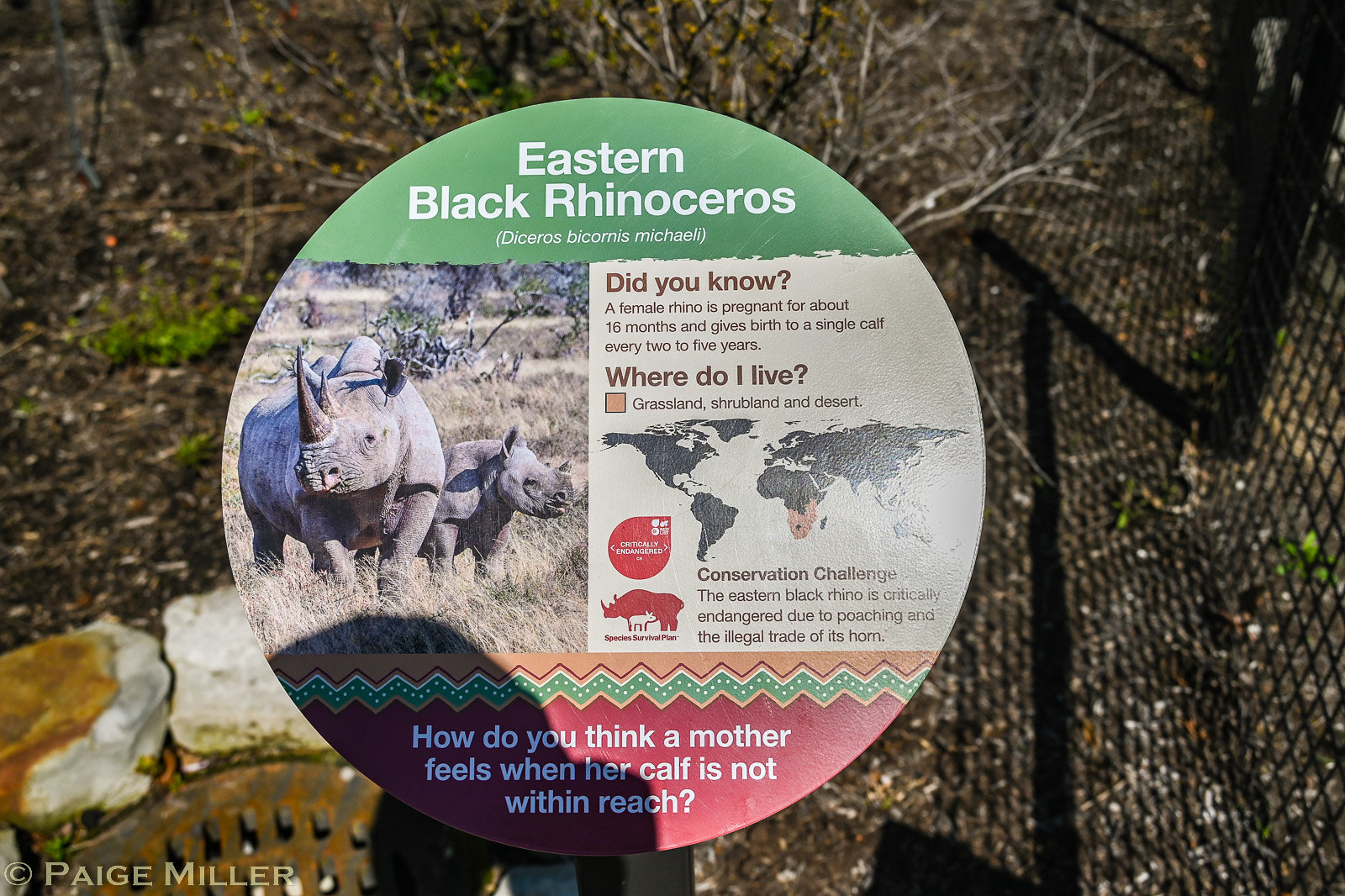The image captures an informative zoo sign set against a backdrop of a dirt area with sparse, twig-like bushes and small white rocks to the bottom left. Visible in the background to the right is a black fence casting a shadow. Central to the image is a circular sign dedicated to the Eastern Black Rhinoceros. At the top of the green sign, the title "Eastern Black Rhinoceros" is prominently displayed in white lettering.

The middle section features a photo of two rhinoceroses in their natural habitat of brown grasslands, flanked on the right by a flat map of the world highlighting the southern regions of Africa where these rhinos are primarily found. Additional information outlines their habitats as grasslands, shrublands, and deserts. The circular sign also includes an educational tidbit: "Did you know a female rhino is pregnant for about 16 months and gives birth to a single calf every two to five years?"

Towards the bottom of the sign, there's a notable conservation message on a red background: "The Eastern Black Rhino is critically endangered due to poaching and illegal trade of its horns." Additionally, it poses a thought-provoking question in white letters: "How do you think a mother feels when her calf is not within reach?"